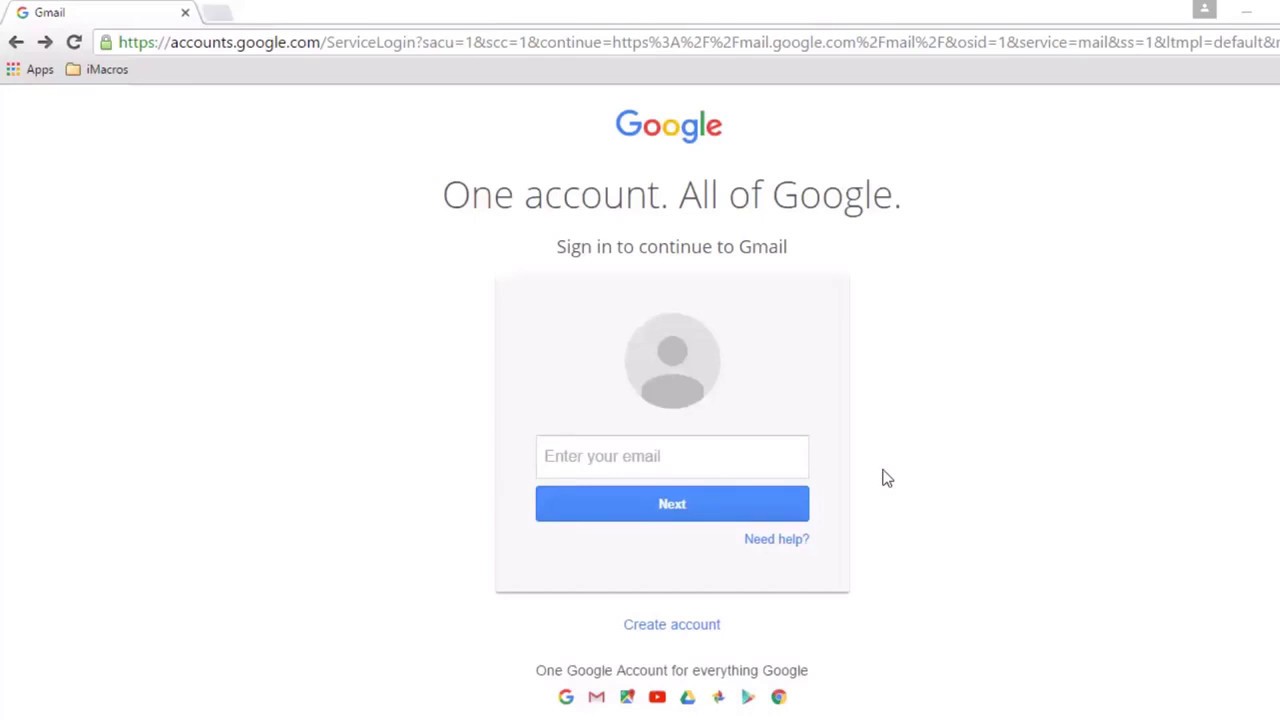The image depicts the sign-in page of Google, accessed via the URL accounts.google.com. The central focus is the Google logo, prominently displayed at the top of the page, featuring its characteristic multicolored letters: the "G" in blue, the first "O" in red, the second "O" in yellow, the second "G" in blue, the "L" in green, and the final "E" in red. Below the logo, the text reads "One account, all of Google," followed by an instruction to "Sign in to continue to Gmail."

The page features a grey and dark grey profile icon above a white input field labeled "Enter your email." Beneath this, a blue "Next" button is prominently displayed. To the bottom right of this button, there is a blue "Need help?" text link. Further down, there is a blue "Create account" text link. Below this link, black text states, "One Google account for everything Google."

At the bottom of the page, icons representing various Google services are displayed, starting with the classic Google "G" in red, yellow, green, and blue. Following icons include Gmail (red and white), Google Maps (multicolored), YouTube (red and white), Google Drive (multicolored), Google Photos (multicolored), Google Play Store (multicolored), and Google Chrome (multicolored). The entire page is set against a clean, white background, keeping the visual focus on the vibrant colors of Google's branding and service icons.